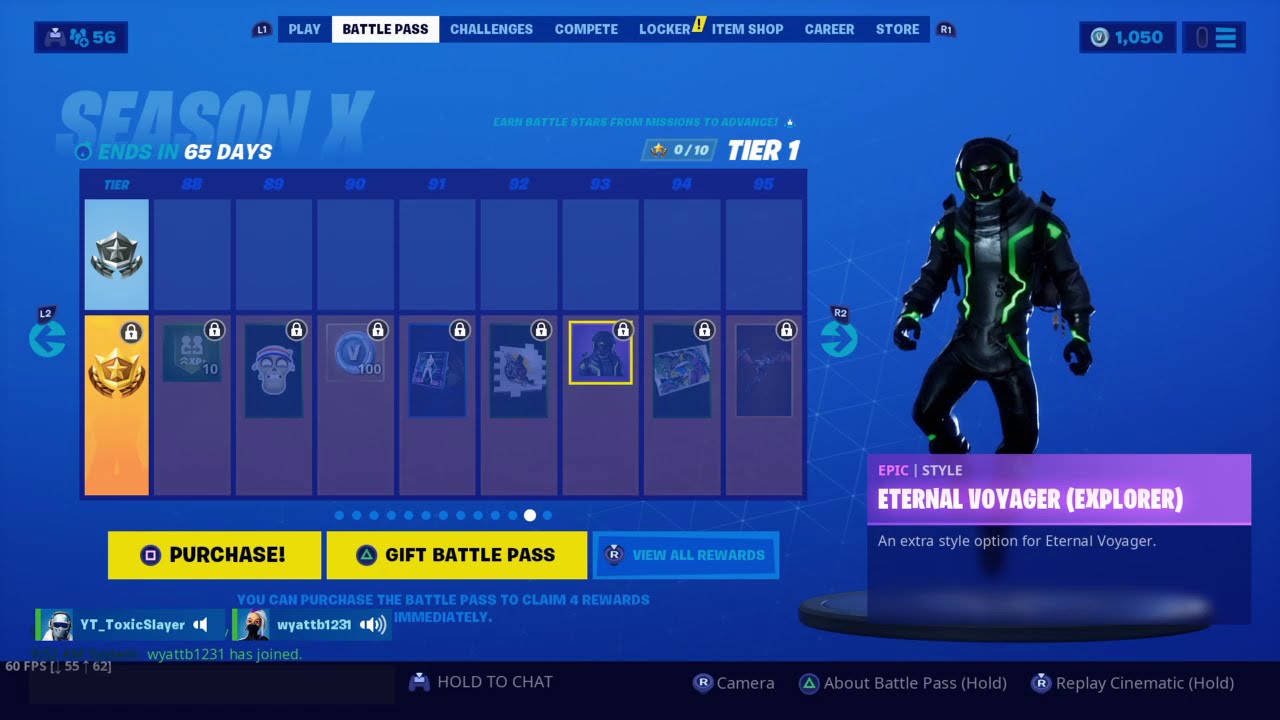The image depicts a detailed screenshot of the Battle Pass screen from the video game Fortnite, specifically for Season X. Dominating the screen is a blue background with a long blue bar at the top displaying various tabs: Play, Battle Pass (selected), Challenges, Compete, Locker, Item Shop, Career, and Store. The text "Season X" is prominently featured near the top, indicating the current season. Below, it notes that the season ends in 60 or 65 days. 

The main focus of the screen is a rectangular box with a series of locked rewards, including silver and gold icons, and a specific section highlighting Tier 1. Additional options invite players to "press the square button to purchase" and "press the triangle button to gift Battle Pass," both on a yellow background with dark blue or black letters. 

On the right side of the screen, a striking black character is displayed, wearing a helmet and a black leather jacket adorned with green neon designs, including glowing lines near the zipper and helmet's ears and eyes. The character is identified as "Eternal Voyager Explorer," with a purple background stating "Epic Style" and "An extra style option for Eternal Voyager." Two usernames, BT Toxic Slayer and Wyatt B1231, are visible in blue letters, likely indicating the current players. Lastly, a small silver coin icon signifies the currency of 1050, situated next to a blue hamburger menu icon.